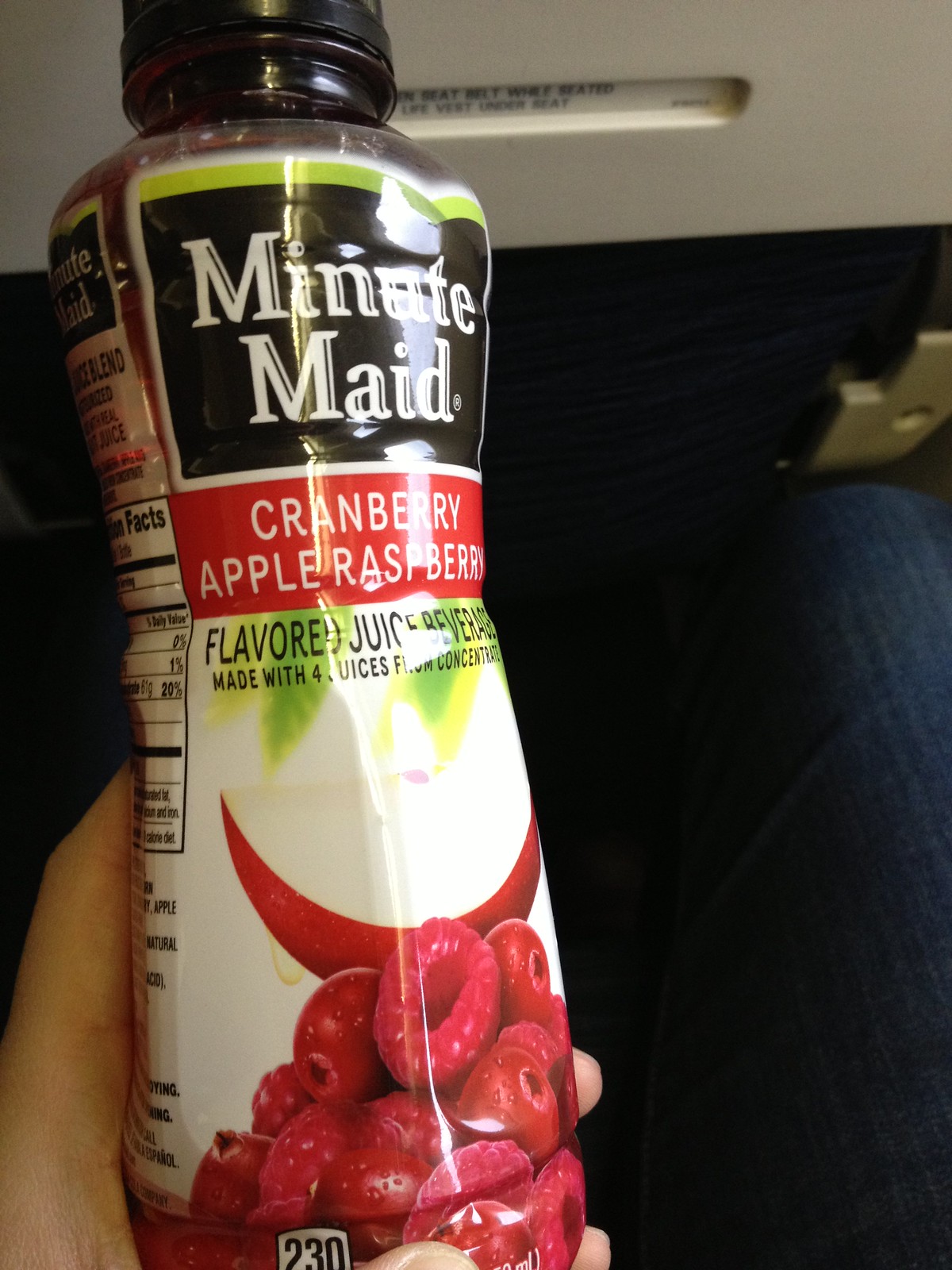This image captures a bottle of Minute Maid juice being held by a person with a fair complexion. The Minute Maid logo, a square black label with the brand name in white letters, is prominently displayed on the bottle. The flavor, a blend of cranberry, apple, and raspberry, is clearly indicated beneath the logo, accompanied by images of these fruits. The bottle is held in a hand that is not gender-identifiable, and the background features the blue fabric of an airplane seat, suggesting the photograph was taken during a flight.